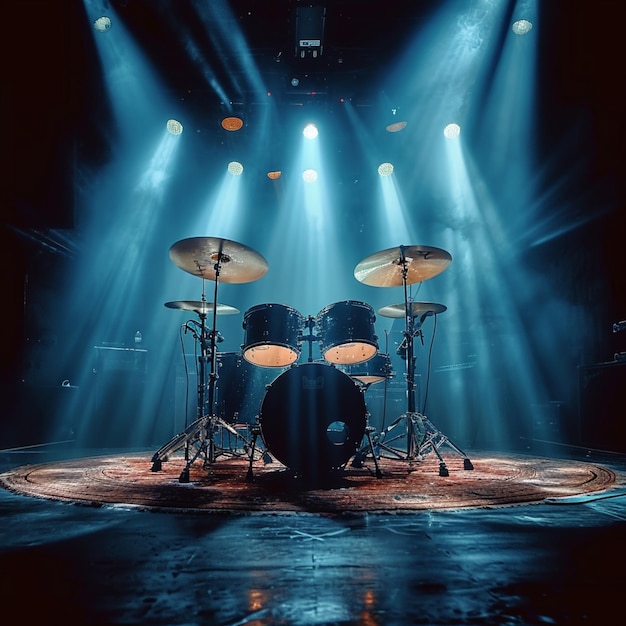In this image, there is a drum set positioned on a stage within a dark room, shrouded in a haze that renders the room’s details indistinct. Bright spotlights with a bluish tint converge on the focal point: a full drum set. The drum set is situated on a round, copper-colored platform that resembles a large rug. The drums are black, with a prominent bass drum in the center flanked by two smaller drums and another drum located at the back, where a drummer would typically be seated. Surrounding the drums are at least four cymbals mounted on stands—two positioned in front and two in the rear. The drum set is also equipped with microphones, suggesting it's prepared for a performance, potentially a legendary drum solo. The setting’s high ceilings and overall dim atmosphere evoke the sense that this is a grand hall or auditorium, with at least 11 spotlights accentuating the instrument in readiness for an anticipated concert.